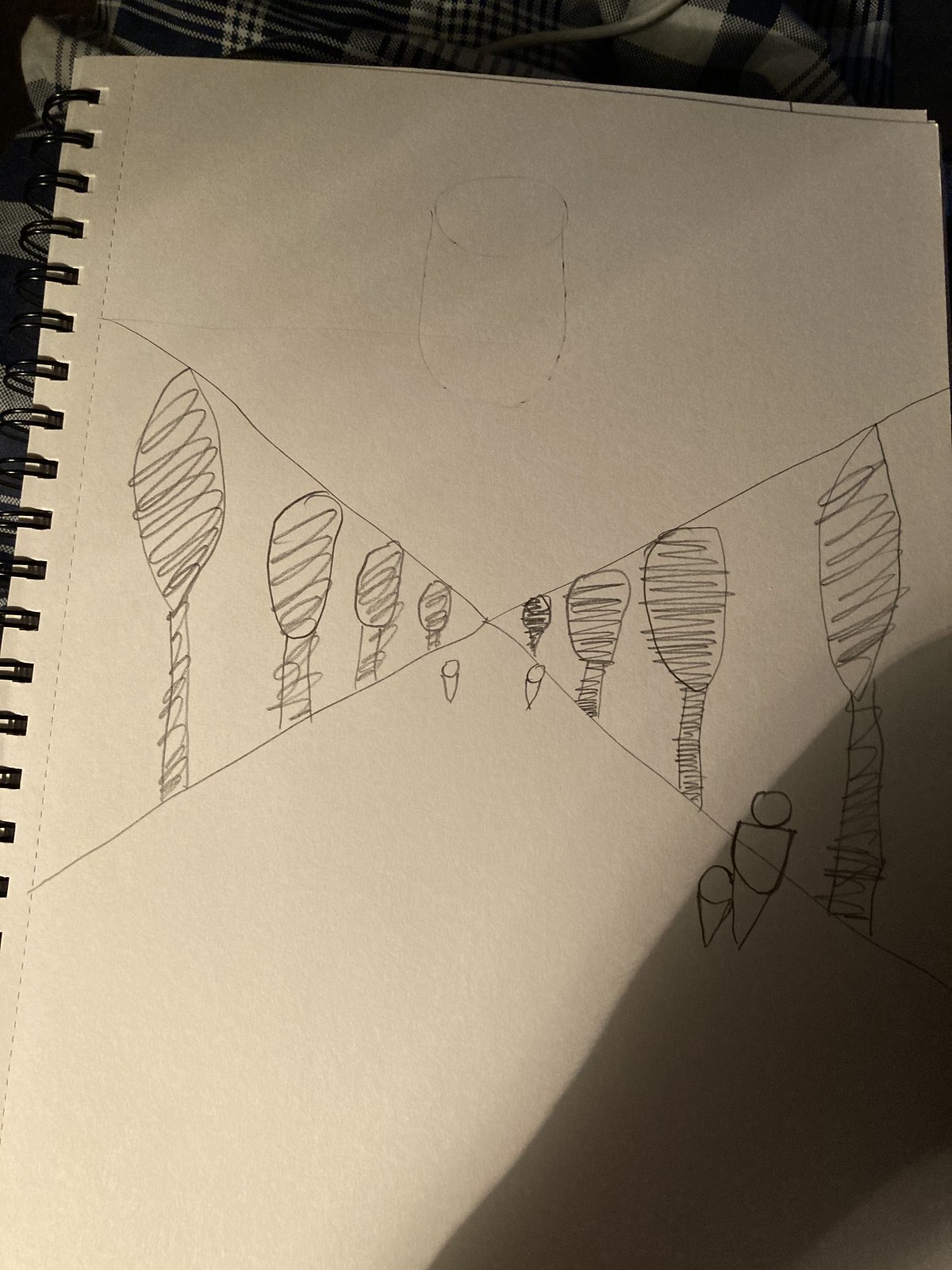This detailed drawing, created using either pencil or pen, initially appears simplistic, reminiscent of a child's doodle. However, upon closer examination, it reveals advanced techniques and thoughtful composition. The piece features a central focal point situated precisely in the middle of the page, representing the horizon. Radiating lines extend from this focal point, guiding the viewer's eye outward. The scene depicts several trees, strategically placed to enhance the sense of depth; the trees closest to the viewer appear larger, gradually diminishing in size as they approach the focal point. This careful arrangement creates a striking perspective, drawing the observer into the artwork's immersive landscape.